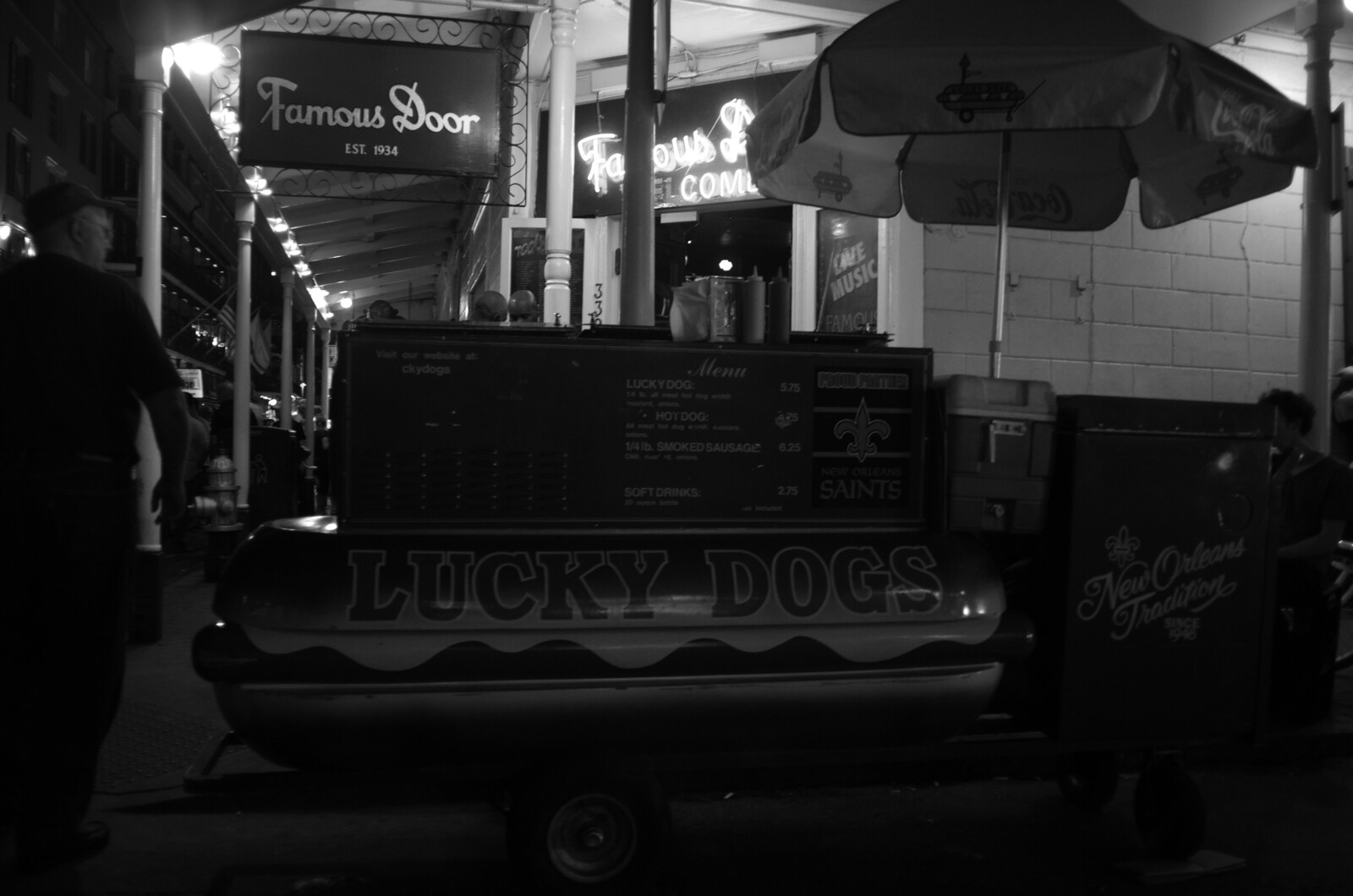In this detailed black and white photo, we see a well-crafted scene centered around a vintage hot dog stand. The stand, in the characteristic shape of a hot dog, prominently displays the name "Lucky Dogs" across its cart, which is equipped with wheels, making it portable. Atop the stand, there’s an umbrella adorned with hot dog illustrations and Coca-Cola branding, providing shelter and attracting the eye.

The background reveals a brick building with a prominent sign, partially covered by the umbrella, that reads "Famous Door, established in 1954." This iconic spot, situated in front of what appears to be a restaurant, is characterized by a covered porch supported by pillars and illuminated by ceiling lights.

Adding to the local charm, the stand is also decorated with New Orleans Saints stickers and a small board displaying its menu items. To the right of the stand, there’s a container labeled "New Orleans Tradition," further emphasizing the cultural relevance of the scene.

In the photograph, a gentleman wearing a cap is seen near the hot dog stand, his dark clothing blending into the grayscale palette. Additionally, on the far left, another man is captured walking toward the restaurant, enriching the lively street ambiance captured in the image.